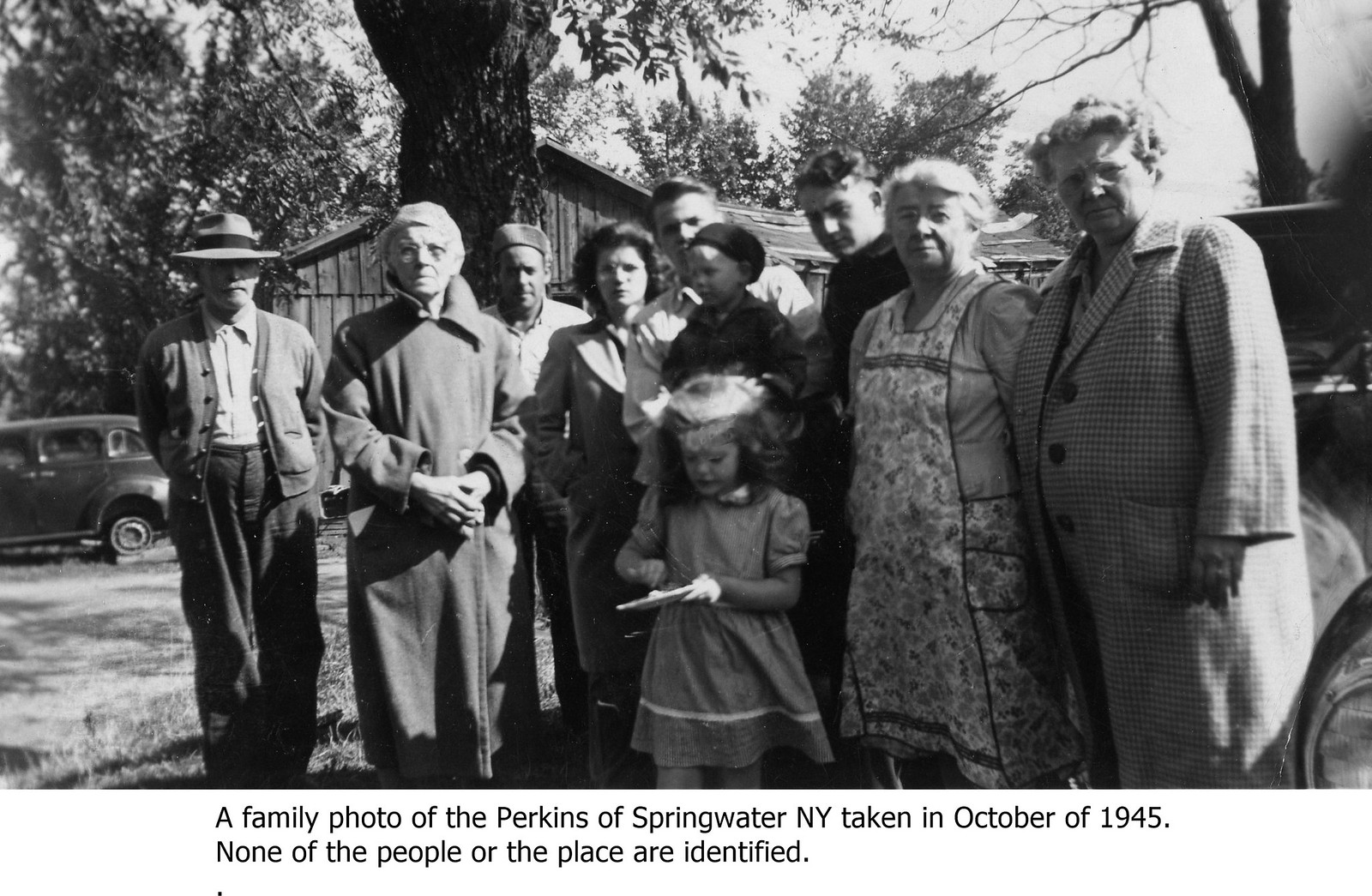The photograph captures a moment from October 1945, featuring a clear and detailed black-and-white image of the Perkins family from Springwater, New York. The group, composed of exactly 10 individuals of varying ages—from a small child being held, likely by his father, to elderly members—stands together posing for the camera. The scene is bathed in natural daylight, suggesting the picture was taken in the daytime. The backdrop includes a vehicle, trees, and what appears to be a house, adding context to the family’s surroundings. A caption beneath the photo reads: "A family photo of the Perkins of Springwater, New York, taken in October of 1945." Although the clarity of the image is excellent, none of the individuals or the specific location are identified.